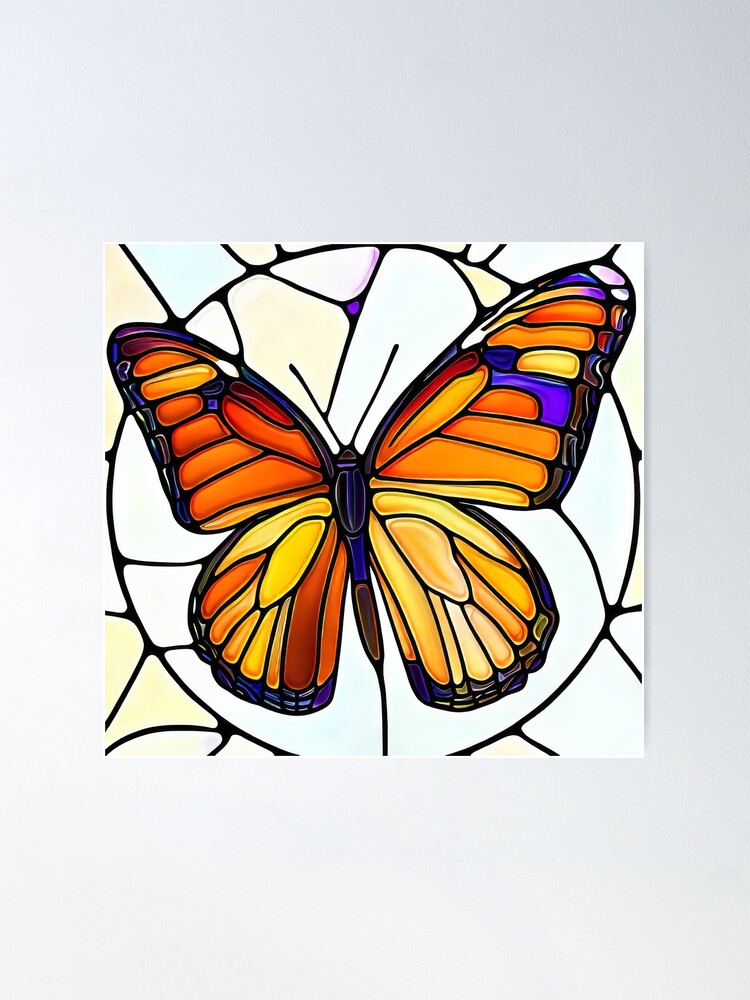The image features a detailed digital rendering of a large butterfly, artistically inspired by stained glass. The butterfly, with its wings spread at a slight angle, showcases a vibrant array of oranges and yellows, accented with rust colors, purples, and subtle blues. Its wings and body are outlined with black borders, mimicking the lead lines typical in traditional stained glass artwork. Surrounding the butterfly is a circular design, broken into uneven pieces featuring varied colors including yellowish tones, light minty green, bluish hues, and some pinkish fragments, all set against a basic grey wall background. These contrasting colors serve to enhance the bold, brilliant colors of the butterfly, making it stand out vividly against the otherwise monochromatic backdrop.